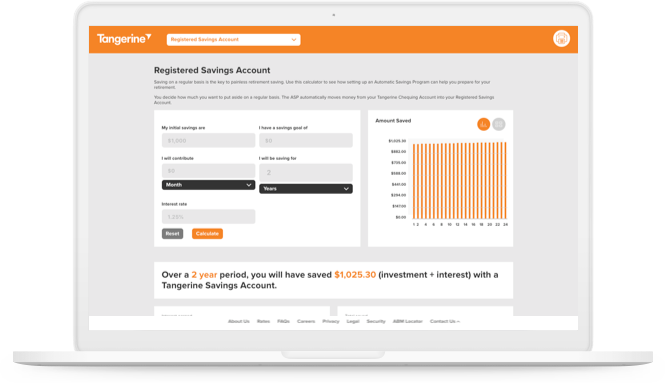**Caption:**

The image displays a webpage of Tangerine, prominently featuring the website's interface. In the top left corner, the word "Tangerine" is visible in bold white text against an orange background that also encompasses the search bar and an icon on the right side. The upper portion and the entire remaining background are light gray. 

Below the header, the text "Registered Savings Account" is clearly stated. Directly beneath this, two sentences provide additional details about the account. The content is further divided into five light gray sections, each containing specific details.

At the center of the image, black buttons labeled "Month" and "Years" are prominently displayed. Accompanying these are a "Reset" button and an orange action button. 

To the right, a chart titled "Amount Saved" is presented, featuring a vertical axis labeled with numbers and a horizontal axis for time, both marked by orange lines. 

The informative text below the chart reads: "Over a two-year period, you will have saved $1,025.30" (with "investment plus interest" in parentheses), followed by the phrase "with a Tangerine savings account." 

At the bottom of the page, there are approximately eight categories listed in very small text, concluding the interface presentation.